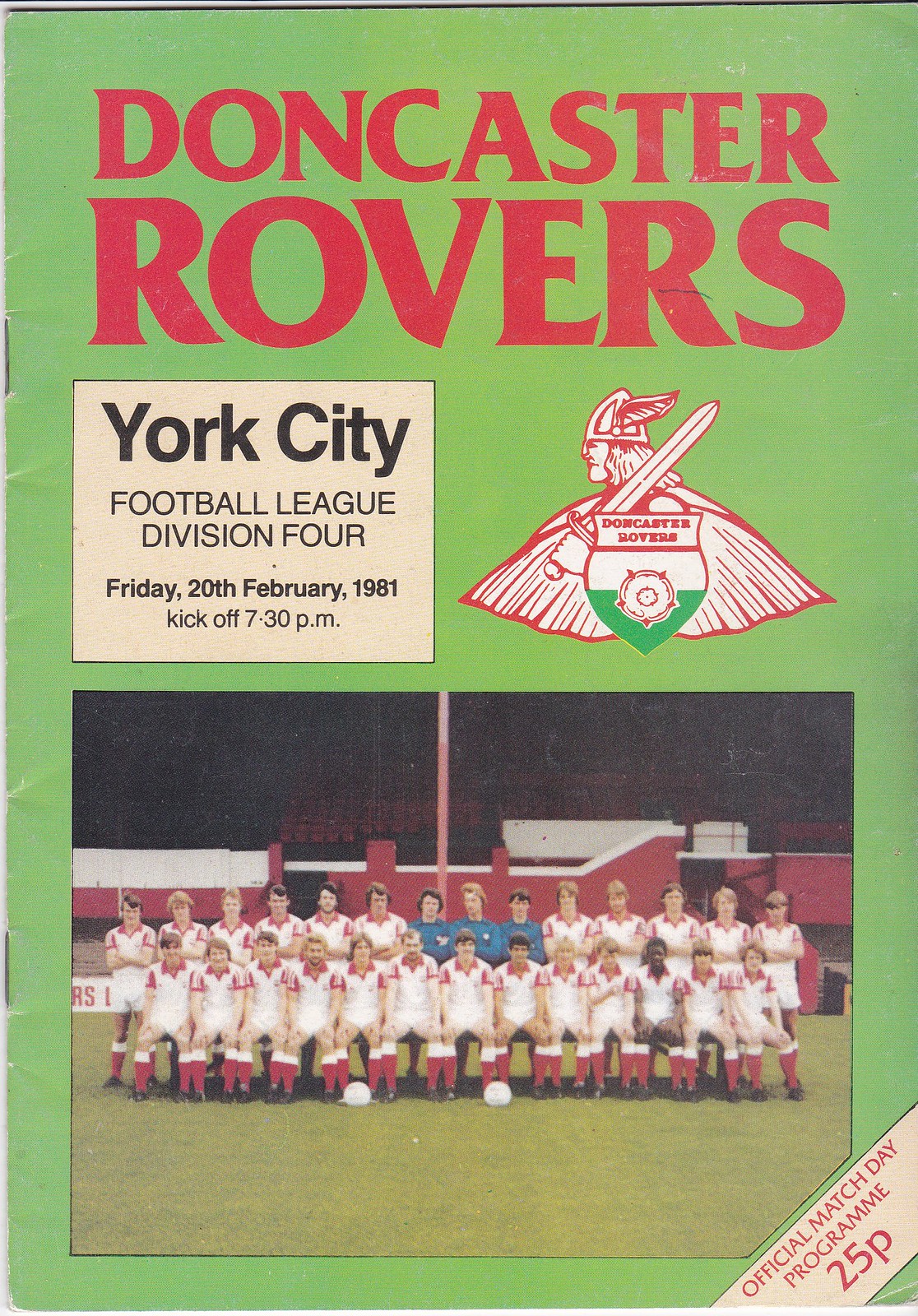The image is a vivid banner for the Doncaster Rovers with a green background. At the very top, bold red letters announce "Doncaster Rovers". Directly below, on the left side, a beige-colored box features black text that reads "York City Football League Division 4, Friday 20 February 1981, kick off at 7.30pm". To the right of this text box is a distinctive decal depicting a Viking in a helmet with a winged decoration, holding a sword over their shoulder. The decal includes a badge with a red outline and a touch of green at the bottom half.

Beneath the decal, a colored photograph showcases the soccer team arranged in two rows, posing on green grass. Most players are dressed in white jerseys with red socks, while three central figures sport blue shirts. Two soccer balls rest on the ground in front of them. The backdrop features a building with red walls and a white upper section. In the bottom right corner, a light cream box with red print states, "Official Match Day Program 25p".